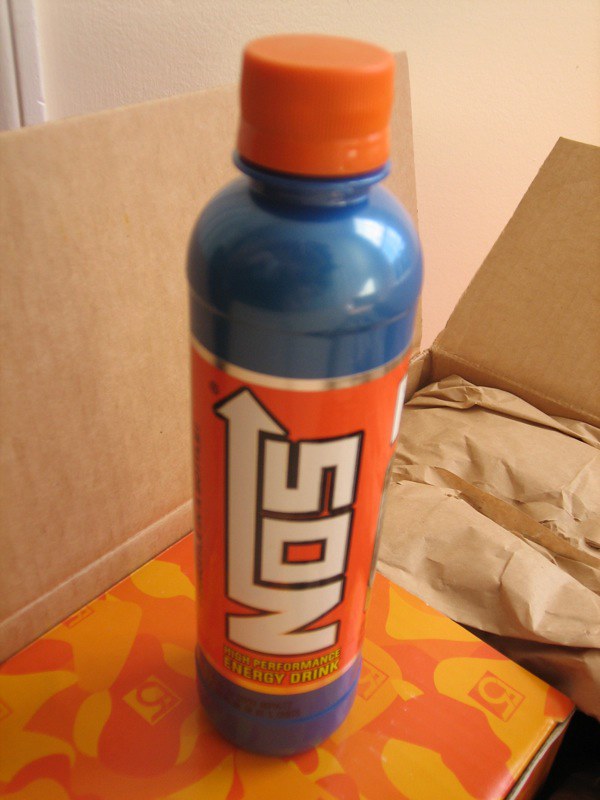This image captures a striking blue energy drink bottle, prominently displaying the brand NOS. The bottle is tall and slender, with an orange cap that appears to be sealed. The label is predominantly orange with white lettering for "NOS," where the 'N' extends into a long arrow that runs underneath the 'O' and 'S.' Below the brand name, in yellow lettering, the words "High-Performance Energy Drink" are clearly visible, along with an indecipherable black stamp near the base of the bottle. The bottle is set against an orange and yellow box that matches its vibrant color scheme. This box, open on two sides and containing some packing paper, suggests that the bottle was originally packaged inside it. The composition centers the bottle on the box, making it the focal point of the photograph.